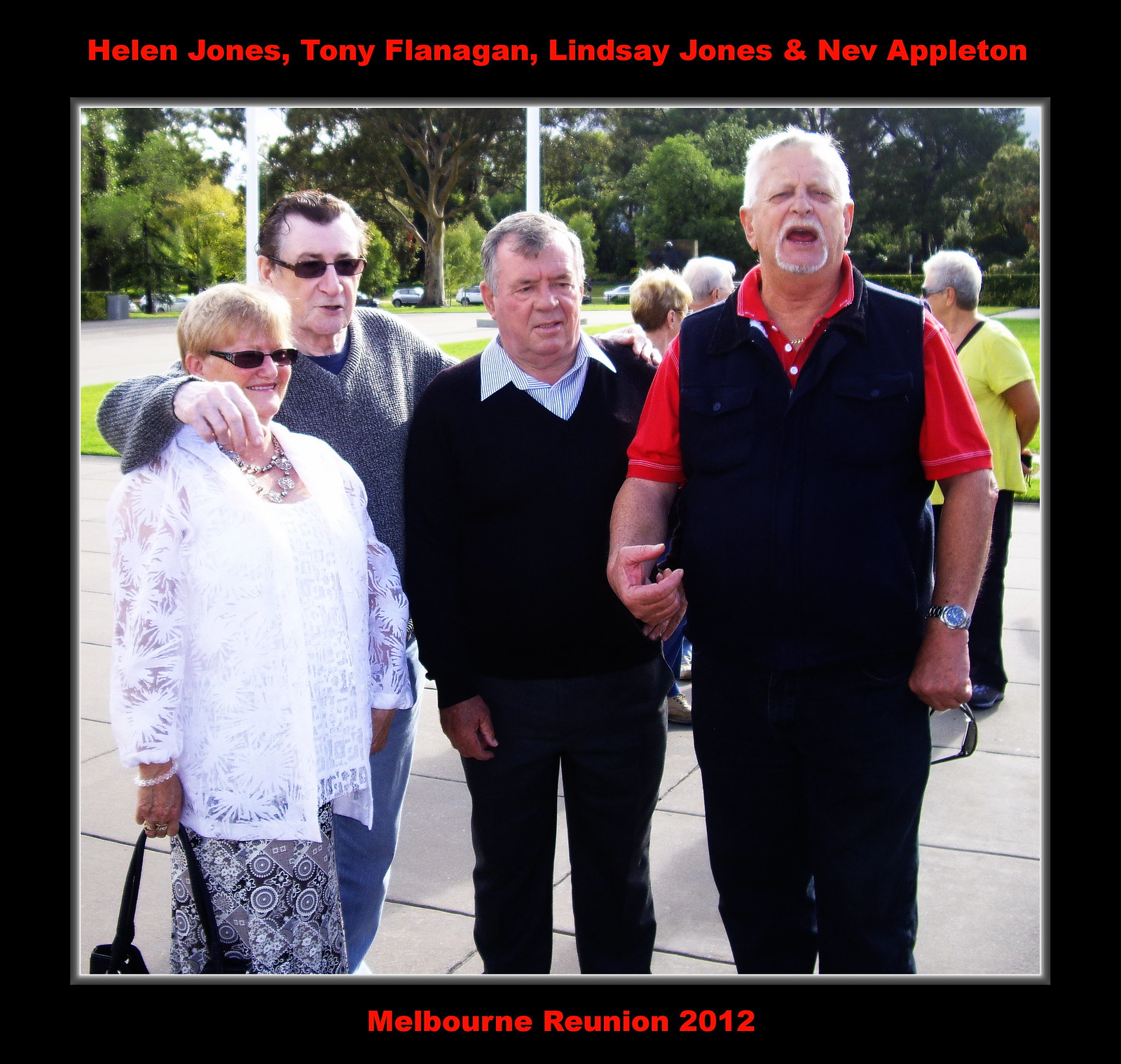The image is a photograph framed by a black border with a silver inner edge. The top border features the names "Helen Jones, Tony Flanagan, Lindsay Jones, and Nev Appleton" in red text, while the bottom border reads "Melbourne Reunion, 2012" in red text. In the foreground of the photograph, four people are posing, all looking forward. The woman on the left is dressed in a white see-through coat over a white blouse, paired with a black skirt adorned with white patterns, and she is holding a black bag. She also has sunglasses on. To her right stands a man in a gray long-sleeve sweater and blue jeans, also wearing sunglasses. Next is another man in a white collared shirt under a black sweater, with black pants. The fourth individual is a man dressed in a red collared t-shirt under a black sweater, also wearing black pants and a watch. All four are standing side by side, clearly captured during a memorable reunion.